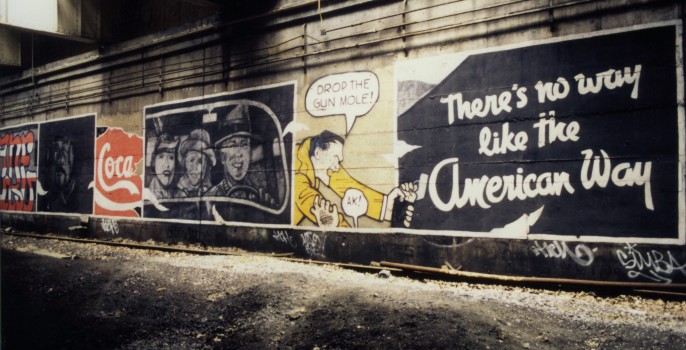In this detailed image, we see what appears to be a subway tunnel adorned with a variety of high-quality murals and advertisements. The floor is covered with gravel, rocks, and other debris, with used and torn-up rails lying against the base of the wall. Above the artwork, cables run along the wall, reinforcing the tunnel environment.

Starting on the left side of the mural array, we see a grim-looking individual adjacent to red and white lettering. Beside this, there is part of a Coca-Cola sign. Central to the wall display, a family portrait from the 1940s shows two ladies and a gentleman in a fedora, all smiling from inside an older car.

Further to the right, the cartoon character Dick Tracy, in his signature yellow coat, is depicted grabbing someone who is partially out of frame. A speech bubble reads, "Drop the gun, mole," while another text overlays this scene with the phrase, "There's no way like the American way." Additionally, the word "ack" appears, indicating a response from the unseen character known as Mole.

Overall, the murals in the tunnel mix classic advertising imagery with comic book art and graffiti, creating a complex and visually engaging scene.